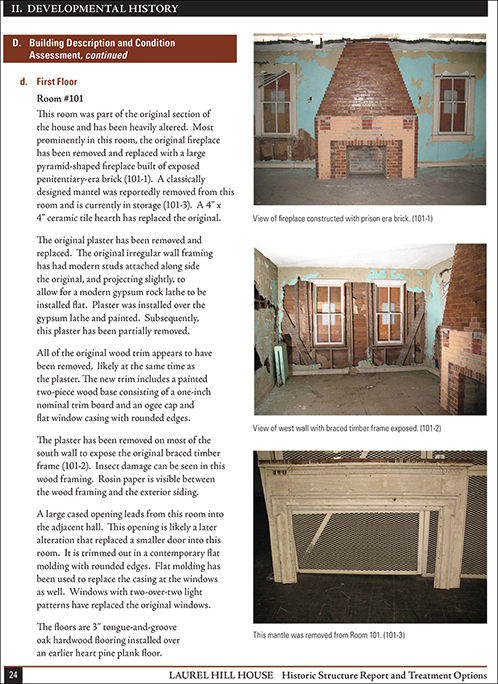The image depicts page 24 of a magazine or brochure focused on the historic Laurel Hill House, providing detailed architectural assessments and renovation suggestions. The title at the top of the page reads "Developmental History, Building Description, and Condition Assessment Continued." The page prominently features three photographs. The first image, located centrally, showcases a brick fireplace within a worn teal-colored room with two windows flanking its sides. Below, the second photograph highlights a dilapidated wall exposing underlying slats between two battered windows. The third image, at the bottom, displays another fireplace, this time of a white hue. Annotations on the page further detail the state of the first floor and discuss renovation options, reinforcing the focus on restoring this historic structure. A legend at the bottom confirms this document as the "Laurel Hill House Historic Structure Report and Treatment Options."